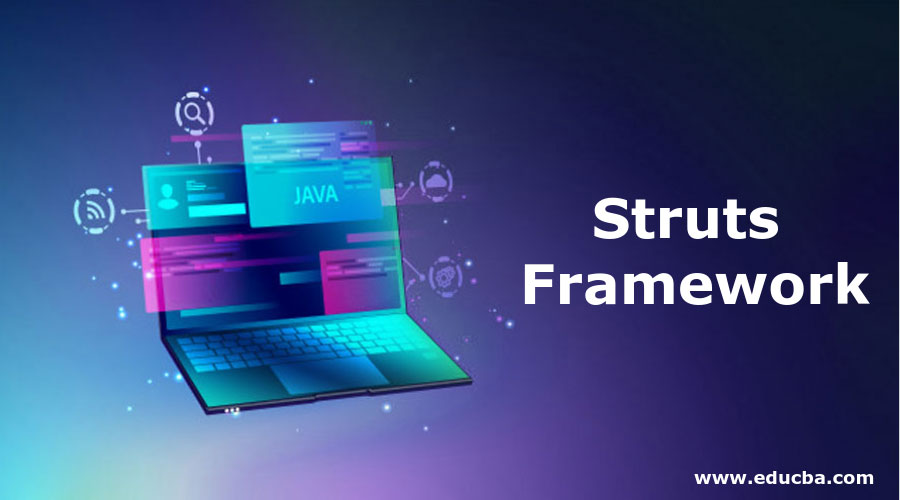The image is a digital ad with a dynamic blue background that transitions from light blue in the bottom left corner to a purple-indigo hue on the right side. Centered on the left part of the ad is a colorful rendering of a laptop, tilted slightly to the right, with a partially visible screen. The keyboard is positioned below while the screen, angled up to the left, features multiple overlapping images. These include a square with the word "Java," a rectangle with a white bar and accompanying text, and various purple and pink elements. Surrounding the laptop are white dots and circles containing icons such as a magnifying glass, a Wi-Fi signal, a cloud, and a couple of gears. In the middle of the ad, bold white sans-serif text reads "STRUTS," with "FRAMEWORK" positioned directly underneath in slightly smaller white letters. The bottom right-hand corner displays the website "www.educba.com" in white text.